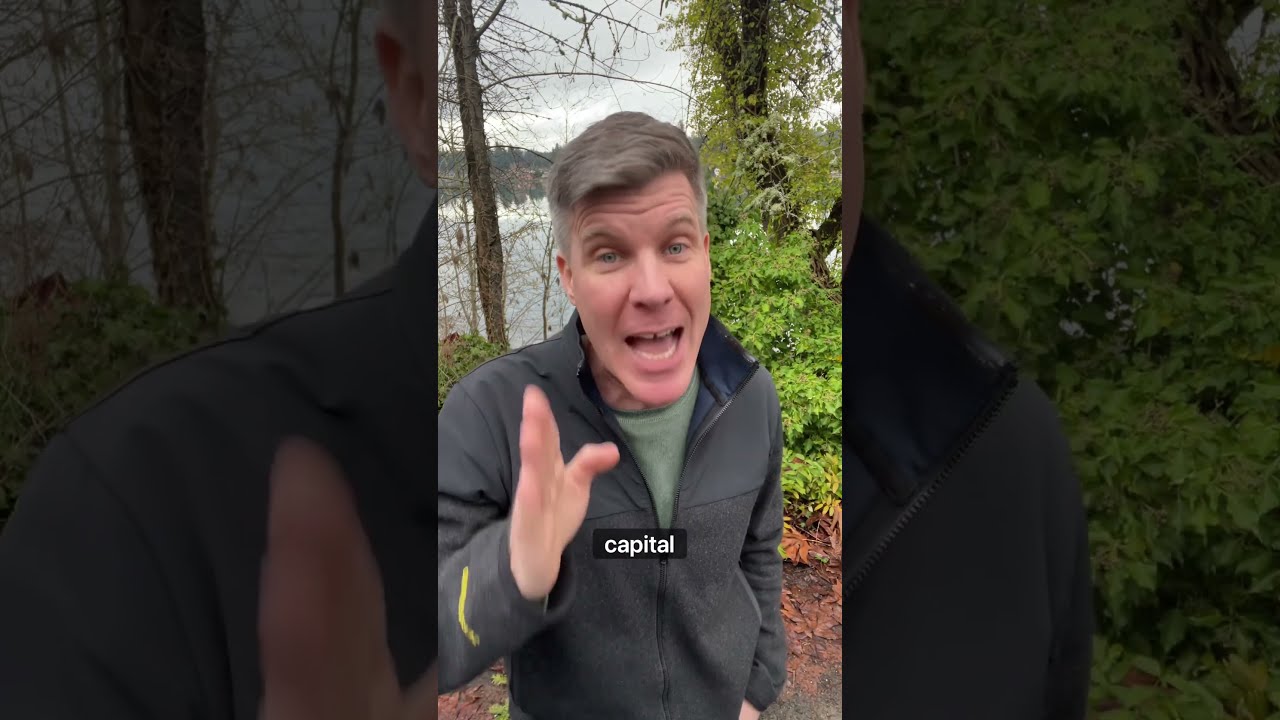In this image, a middle-aged white man stands in a scenic woodland area, speaking passionately into a camera. He appears to be recording an outdoor podcast or video, engaging viewers with his expressive demeanor. The man has short, light brown hair with gray streaks above his ears and a discernible gap between his two front teeth. His forehead shows a few wrinkles, adding to his earnest expression as he holds up his hand, emphasizing a point. 

He is dressed in a gray zip-up sweater with blue lining, layered over a green shirt. Surrounding him are lush green trees, with one prominent tree behind him adorned with ivy. In the background, there is a serene body of water, likely a lake or pond, and further in the distance, rolling hills transition into a mountain range, creating a picturesque backdrop. The overall ambiance suggests he is deeply engaged in discussing an important topic, with the natural environment enhancing the sense of authenticity and tranquility.